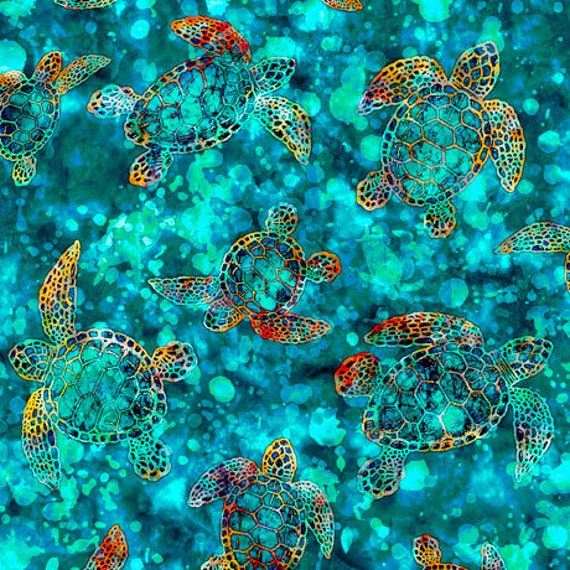In this vibrant square image, a mesmerizing scene of sea turtles unfolds against a dynamic and colorful backdrop. The background is filled with bubbly, light green shapes, interspersed with darker green shades, creating an effect reminiscent of underwater bubbles or a sparkling watery environment. The light greens and teals give the impression of freshness and movement.

Amidst this backdrop, six to seven sea turtles float gracefully in various directions—up, down, left, right, and diagonal. Their shells mirror the background's greenish hues, seamlessly blending with the surroundings. However, the turtles' limbs, highlighted in striking shades of orange and black, stand out and give an impression of luminescence, as though they are subtly glowing.

The turtles vary in size, with some appearing larger or smaller than others. This variation enhances the sense of depth and perspective within the image. The lower corners of the image feature partial turtle figures, while more complete and detailed depictions float centrally. Altogether, the image captures a whimsical underwater ballet of sea turtles amidst a beautifully rendered, aquatic bubble world.